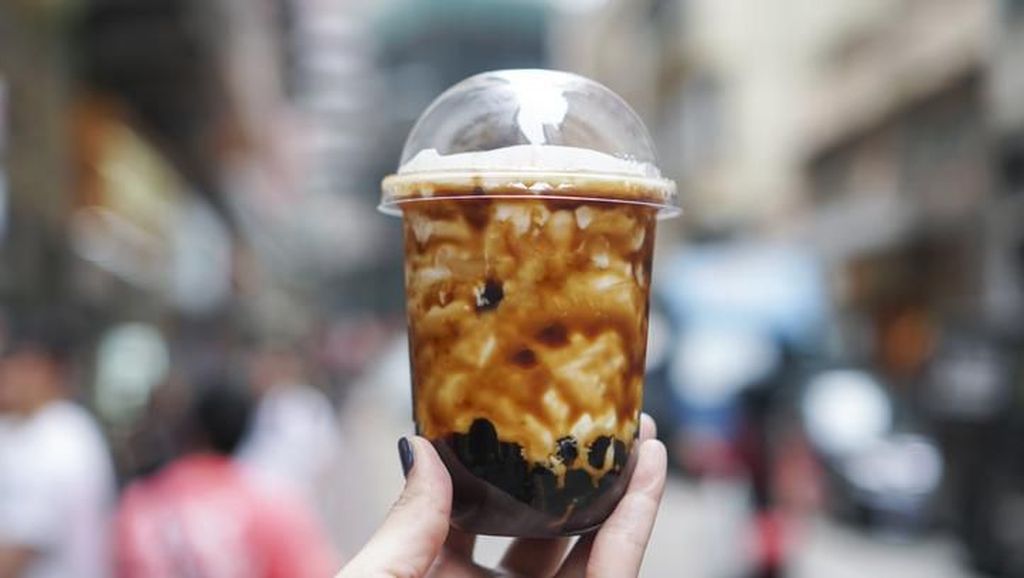A detailed photograph captures a fancy coffee drink held by a woman with black fingernail polish. The drink, in a clear plastic cup with a rounded dome lid, appears composed of layers of white foam, caramel glaze swirls, and chocolate or berry-like elements at the bottom. Light reflecting off the dome lid adds a shiny white effect. The background features a heavily blurred urban scene filled with indistinct buildings and pedestrians, creating a strong bokeh effect that keeps the focus on the intricate details of the drink and the polished nails of the female hand holding it.